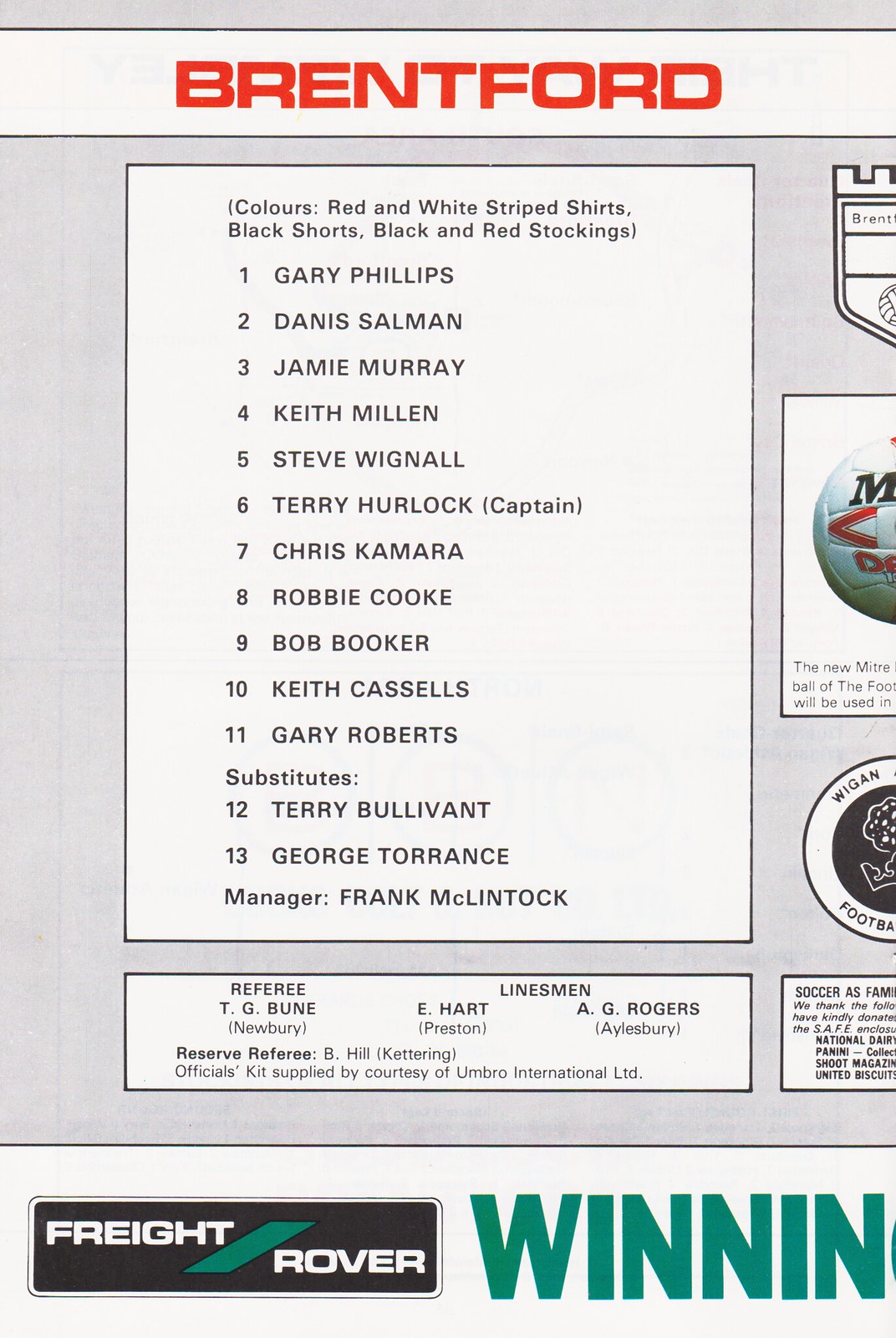The image depicts a detailed roster and game information for a soccer match. At the top, "Brentford" is prominently displayed in bold red letters. Below, it lists the team's colors as red and white striped shirts, black shorts, and black and red stockings. The image displays a white square set against a gray background, containing a list of 13 player names and their numbers: 1. Gary Phillips, 2. Dennis Salman, 3. Jamie Murray, 4. Keith Millen, 5. Steve Wignall, 6. Terry Herlock (captain), 7. Chris Camara, 8. Robby Cook, 9. Bob Booker, 10. Keith Cassells, and 11. Gary Roberts. Substitutes listed are: 12. Terry Boulevant and 13. George Torrance. The manager is noted as Frank McClintocks. Additional information includes details about the match officials: Referee T.G. Boone from Newberry, linesmen E. Hart from Preston and A.G. Rogers from Aylesbury, and reserve referee B. Hill from Kettering. The bottom part of the image also contains the text "Freight Rover winning," rounding out the comprehensive match overview.